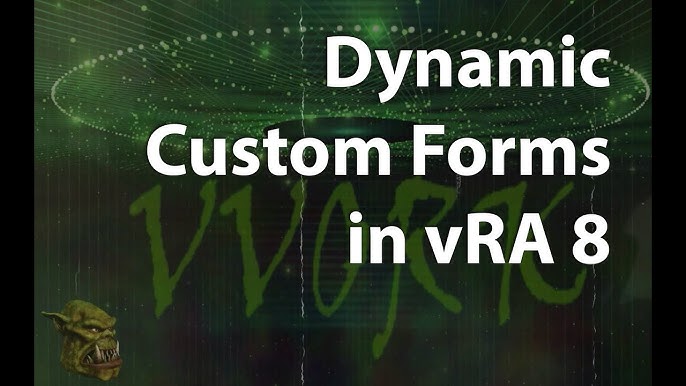The image appears to be a graphic design, possibly a PowerPoint slide, with a green and white background featuring an outer space theme filled with abstract lines and circular shapes. At the top center, three lines of white text read: "DYNAMIC" on the first line, "CUSTOM FORMS" on the second line, and "INVRA8" on the third line. The background has a green watermark that spells out "VVORK" in a dripping font. Vertical black borders run along the left and right sides of the image. The bottom left corner depicts a menacing, ogre-like creature with green skin, a triangular head, pointy ears, and sharp, protruding teeth. The creature has an underbite and large, gruesome features, resembling a monstrous version of Shrek. The central part of the background includes white dots forming a circular pattern that might suggest a spaceship-like design. The colors in the image are mainly black, white, green, and yellow.